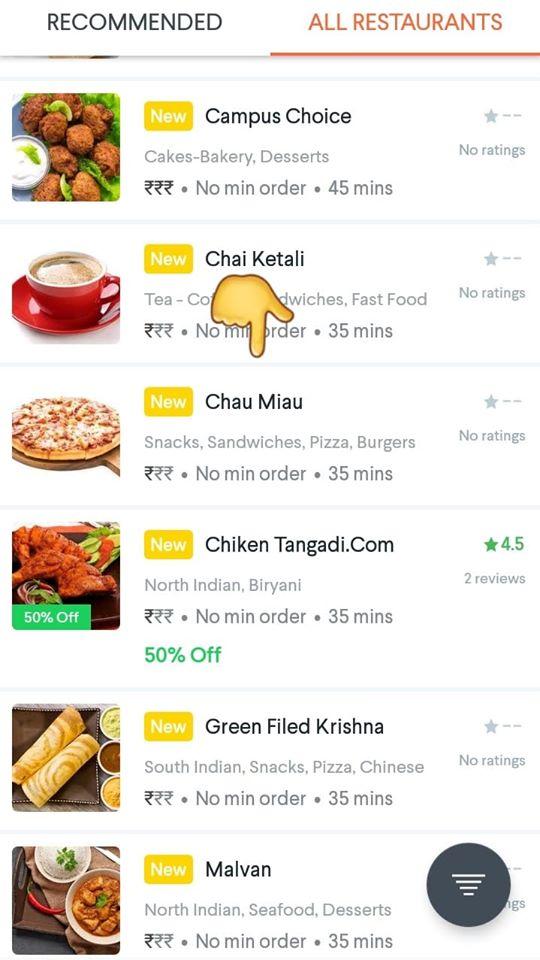The image is a portrait-format menu featuring an assortment of food items and promotions. At the top left corner, the word "Recommended" is prominently displayed in black text, while "All Restaurants" appears in red on the top right, underscored by a red line. The currency, depicted with two parallel lines and a checkmark-like symbol, is unfamiliar.

The menu is cluttered with multiple thumbnail images of meals listed on the left side. The top item is labeled "Campus Choice" with the word "New" highlighted in yellow. It showcases a dish consisting of cooked balls surrounded by green lettuce and accompanied by a white sauce.

The second item is a beverage, possibly tea, coffee, or hot chocolate, served in a red cup, and is named "Chai Ketali". 

The third item, "Chow Meow", includes a list of offerings such as snacks, sandwiches, pizza, and burgers, with a thumbnail image of a pizza.

Next, "Chicken Tangadi.com" is displayed with a picture of fried chicken wings and a promotional note indicating "50% off" in green text, along with a rating of 4.5 stars.

Following that, "Green Filled Krishna" features an image of some type of rolls.

Lastly, "Malvan" highlights North Indian seafood and desserts with an image showing two bowls – one filled with rice and the other with curry.